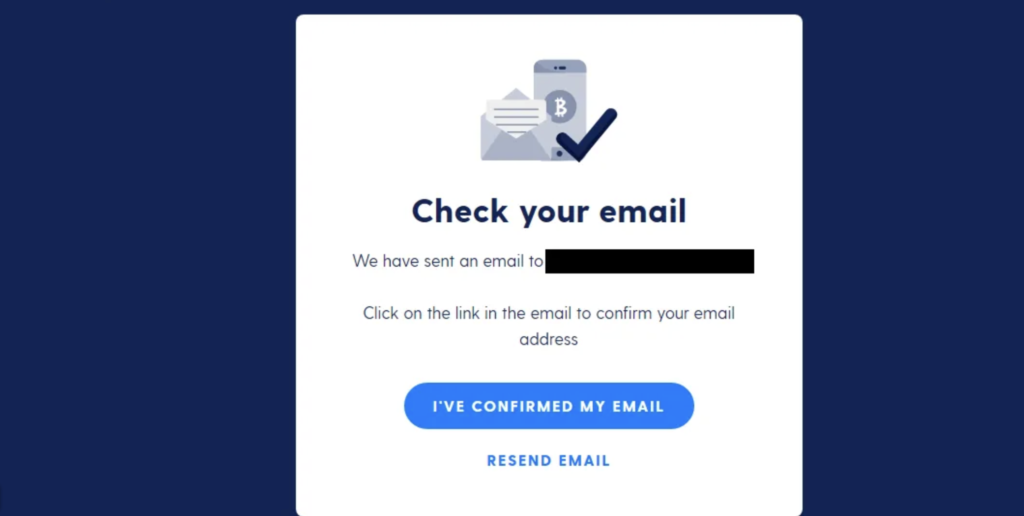The image features a dark blue background with a prominent white box centered within it. Inside the white box, at the top center, there is an illustration of an envelope with a piece of paper protruding from it. Behind this envelope is another envelope marked with a circle containing a white bead and a large blue check mark.

In large, dark blue letters at the top, the text reads, "Check Your Email." Below this, in lighter blue letters, it says, "We have sent an email to," followed by a redacted email address. It continues with, "Click on the link in the email to confirm your email address."

Towards the bottom of the white box, there is a large blue button with white text that states, "I've confirmed my email." Beneath this button, in blue text, is the option "Resend email."

The overall layout emphasizes the importance of checking your email inbox and confirms the receipt of an email requiring the user’s action to confirm their email address.